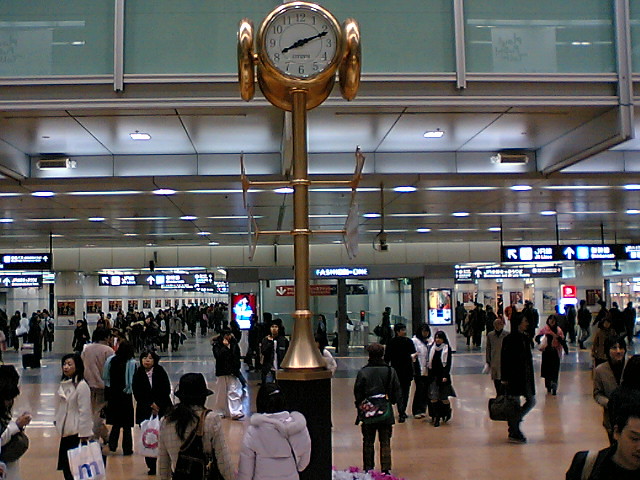This is a detailed picture of the interior of a large train station, characterized by its bustling activity and architectural features. The focal point of the image is a prominent golden clock tower situated in the middle of a spacious, open lobby. This elegant timepiece features a square black plinth, a circular brass base, and a 10-foot brass pipe extending upwards to support four circular clocks, each facing a different direction. The clock facing the camera displays the time as approximately 8:12, with a white face and black hour and minute hands. Surrounding the clock tower, numerous people, many of whom appear to be of Asian ethnicity, are seen walking through the station. Overhead signs, presumably directing travelers to various rail lines, are visible but the text is overexposed and illegible. Some of these signs also feature Asian script, further indicating the location's cultural context. The image captures the dynamic atmosphere of the station with its steady flow of passengers and intricate design elements.